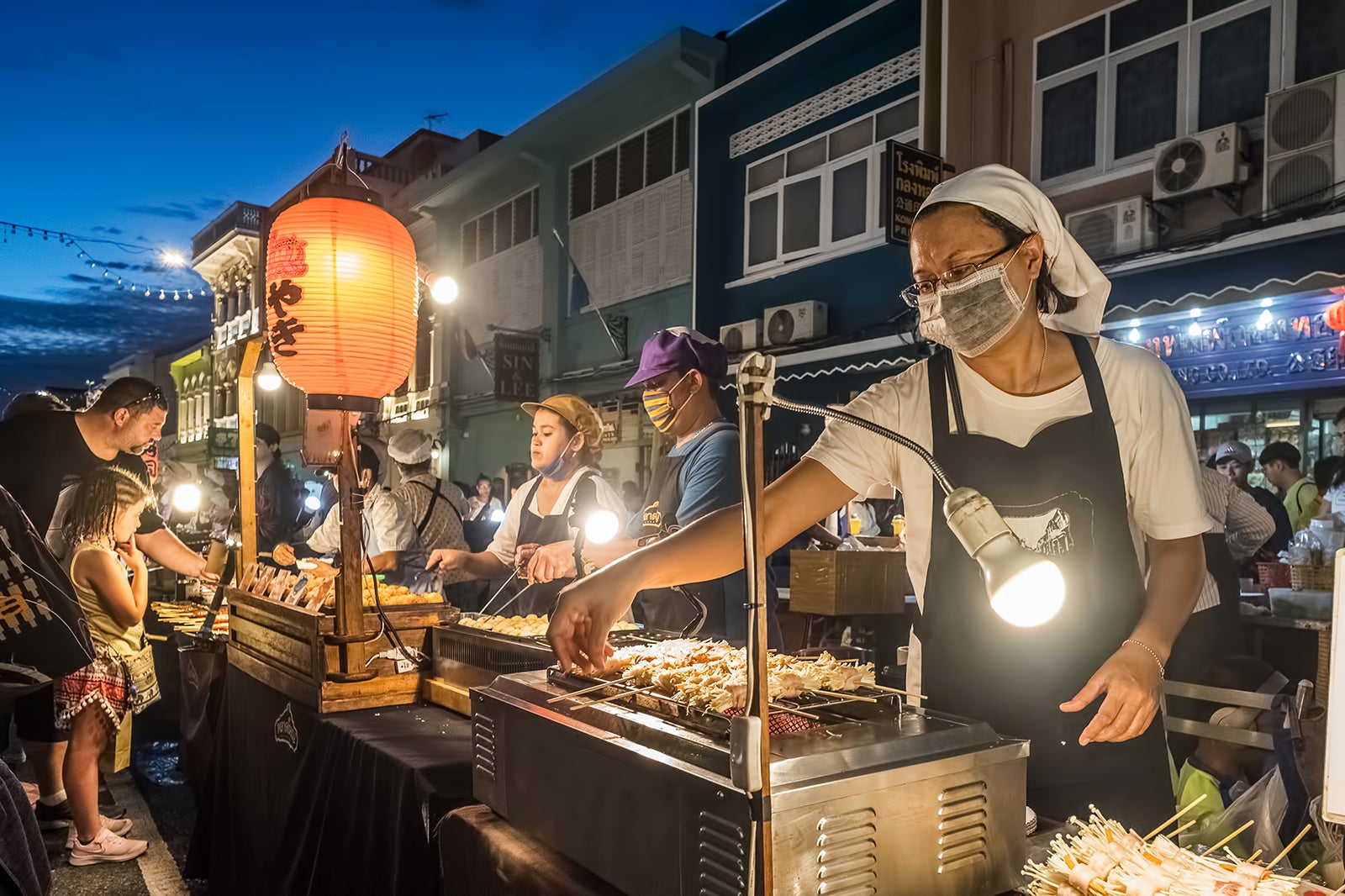This image captures a vibrant Asian street food market scene at dusk, transitioning into night. The photograph, taken with a high-quality camera, showcases a bustling marketplace where various food vendors, some wearing masks, are diligently grilling and frying an array of dishes. Among the foods being prepared, grilled chicken and squid are prominent. The setting is illuminated with lights and features a distinctive paper lantern adorned with Asian writing, which adds to the cultural ambiance. The background reveals several buildings, likely a mix of restaurants, business offices, and apartments, some with visible air conditioning units. On the left side of the image, a little girl with braided hair and a man with sunglasses atop his head can be seen examining the street food offerings. The market is filled with a diverse crowd, both locals and visitors, contributing to the lively atmosphere of what appears to be a typical evening outing in an Asian neighborhood.